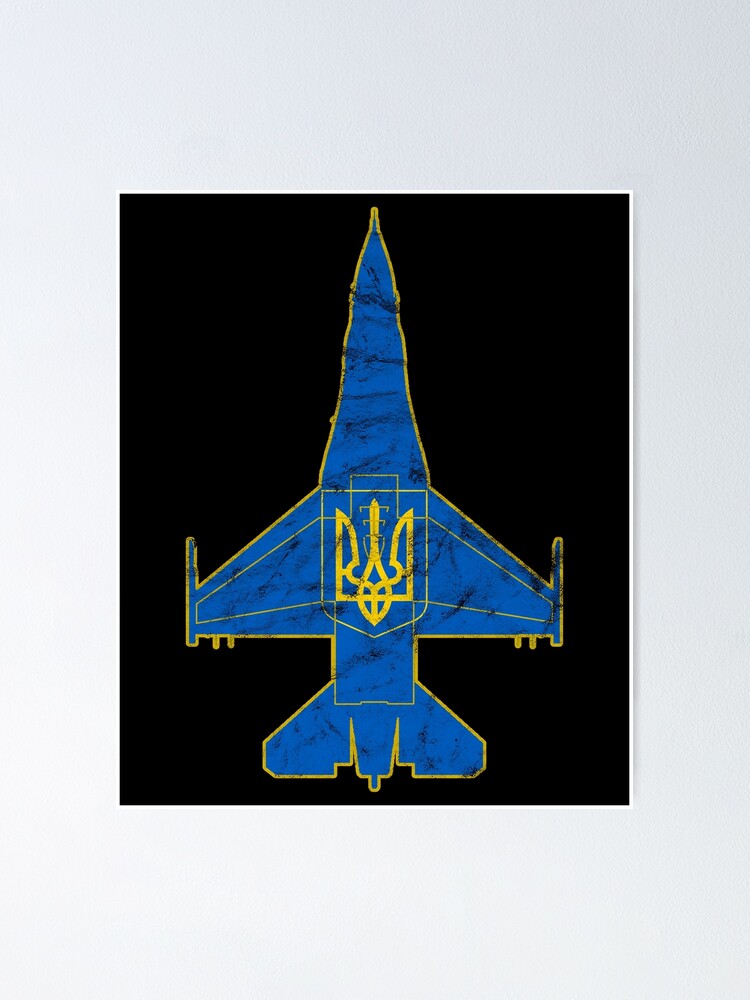The image is a detailed, vertically-oriented drawing or painting of a futuristic fighter jet, centrally placed within a light gray vertical rectangle that has a black background. The jet is depicted from a top view, with a sharp, needle-like nose at the top of the image. The cockpit area is positioned at the front of the plane, and mid-section wings extend outward, just below the center of the black rectangle, featuring cylindrical protrusions that resemble missiles at their tips. Smaller rear wings and accompanying engines are visible towards the back.

The body of the jet is primarily blue, with black streaks interspersed throughout, adding texture. Yellow outlines trace the shape of the jet, and additional yellow and gold lines and shapes adorn its interior, contributing to a layered, design-rich appearance. In the middle section, there's a yellow symbol that appears to consist of an R on the left, an S on the right, and a shape resembling a tennis racket or shield in between, with curvy, bird-like wings extending from it. The overall look is intricate and dynamic, with various lines and shapes suggesting a complex, layered structure.